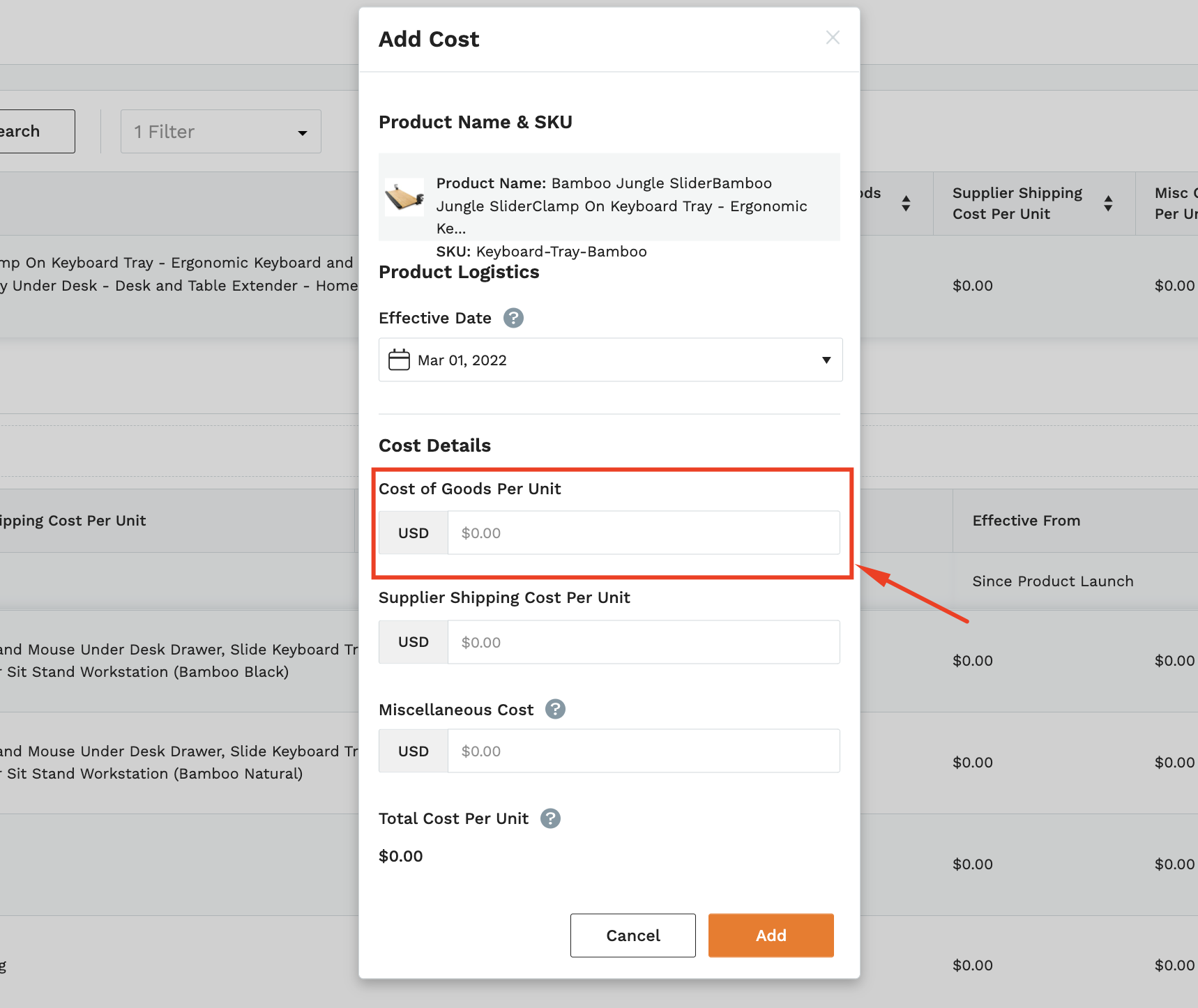The image caption cleaned up and reformulated into a detailed descriptive caption is as follows:

"The image displays a popup box titled 'Add Cost' at the top. It includes fields for product name and SKU. The product listed is 'Bamboo Jungle Slider Bamboo' with the SKU 'Keyboard Tray Bamboo'. To the left of these fields, there is a thumbnail image of the product. Below it, the box lists 'Product Logistics' and 'Effective Date', which is set to March 1st, 2022, with a dropdown menu. 

Further down, under 'Cost Details', there are several fields: 'Cost of Goods Per Unit' showing $0.00, 'Supplier Shipping Cost Per Unit' also showing $0.00, 'Miscellaneous' $0.00, and 'Total Cost Per Unit' at $0.00. There is a red box with an arrow pointing to the cost details. At the bottom right of the popup box, there are options to either 'Add,' indicated by an orange dollar box, or 'Cancel' to exit.

In the background, the interface displays a search bar and a filter section with one active filter. The layout is uniform, with a header followed by product information in a table format. This table reflects the same cost information from the popup box: 'Supplier Shipping Cost' as $0.00. The second product listed is the 'Mouse Under the Desk Drawer,' which also shows $0.00 in both cost columns. The products differ in their color descriptions, with one being 'Natural' and the other 'Bamboo'."